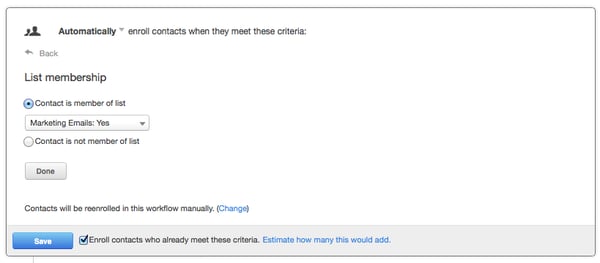This image depicts a status page for a website, likely part of a marketing automation tool designed for business use. At the top of the page, a heading in black and white reads, "Automatically enroll contacts when they meet these criteria." Directly beneath it, a "Back" option is visible for navigation purposes. Below the "Back" option, another section title says "List Membership" in black and white text.

The main content area includes a selectable round button next to the text, "Contact is a member of this list." This option seems to be currently active. Below this, a drop-down menu labeled "Marketing Emails" is set to "Yes." 

Further down, another selectable option reads "Contact is not a member of the list," providing an alternative criterion for contact enrollment. Beneath this, a "Done" button is present, signifying the end of selectable criteria. Below the "Done" button, there's an important note, "Contacts will be re-enrolled in this workflow manually."

At the very bottom of the page, two buttons are visible. The first is a blue clickable "Save" button, and next to it is a note that says, "Enroll contacts who already meet these criteria. Estimate how many this would add."

This detailed layout suggests the page facilitates setting up automated criteria for enrolling contacts into different workflows, likely to streamline email marketing efforts.